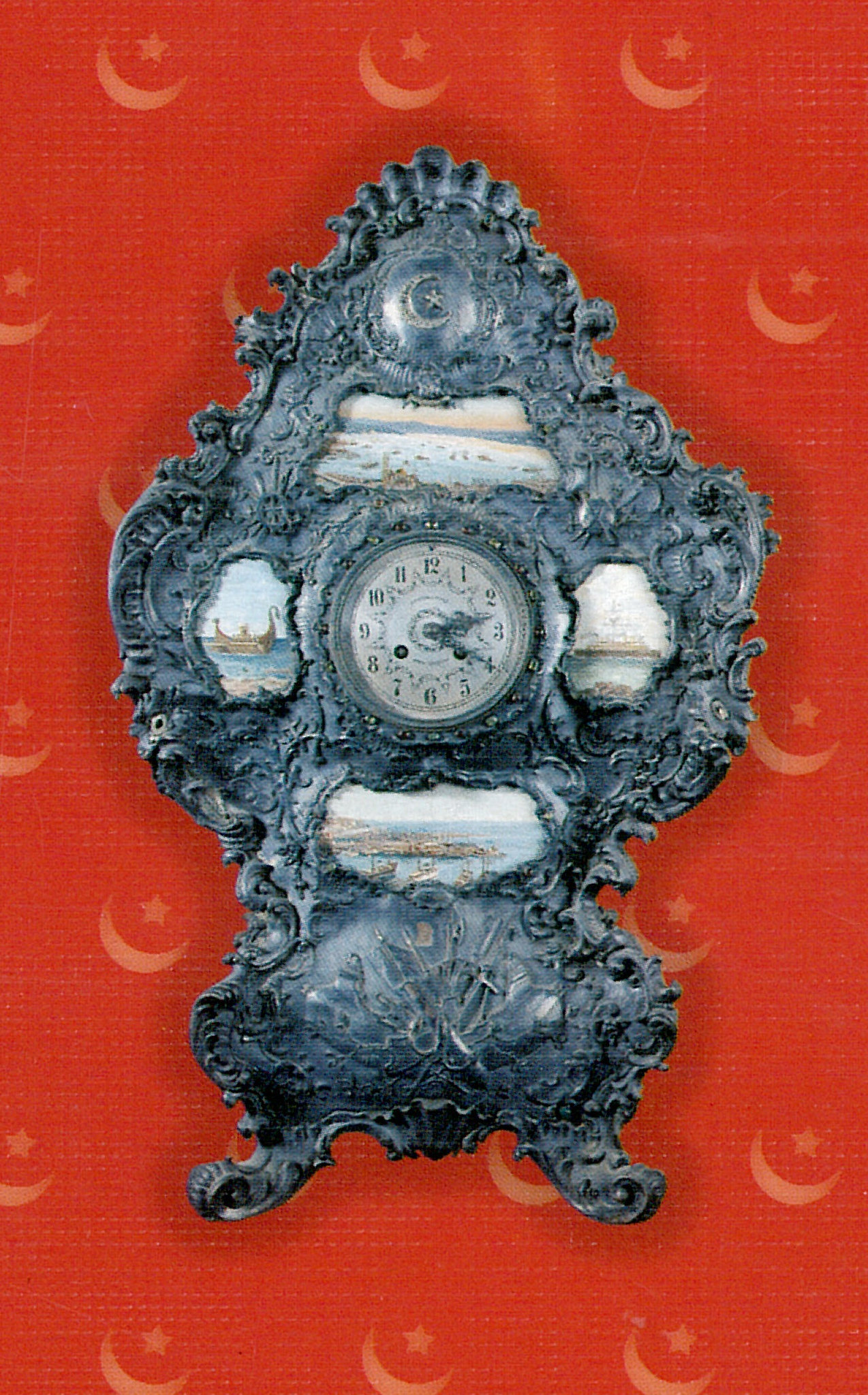This image features a clock set against a vibrant red background adorned with a repeating pattern of white crescent moons and five-point stars. The clock itself is circular, with an off-white or light gray face and black hands, indicating the time as 2:20. Surrounding the clock is an elaborate, black, cast-iron structure that resembles a bear standing upright. The structure includes legs on either side and intricate carvings at the top, bottom, left, and right. Within this decorative frame, there are small, detailed artworks that depict scenes of a beach and waterway with sailboats. The entire scene is visually busy and meticulously detailed, giving the impression of a heavy, dense, and ornate piece.